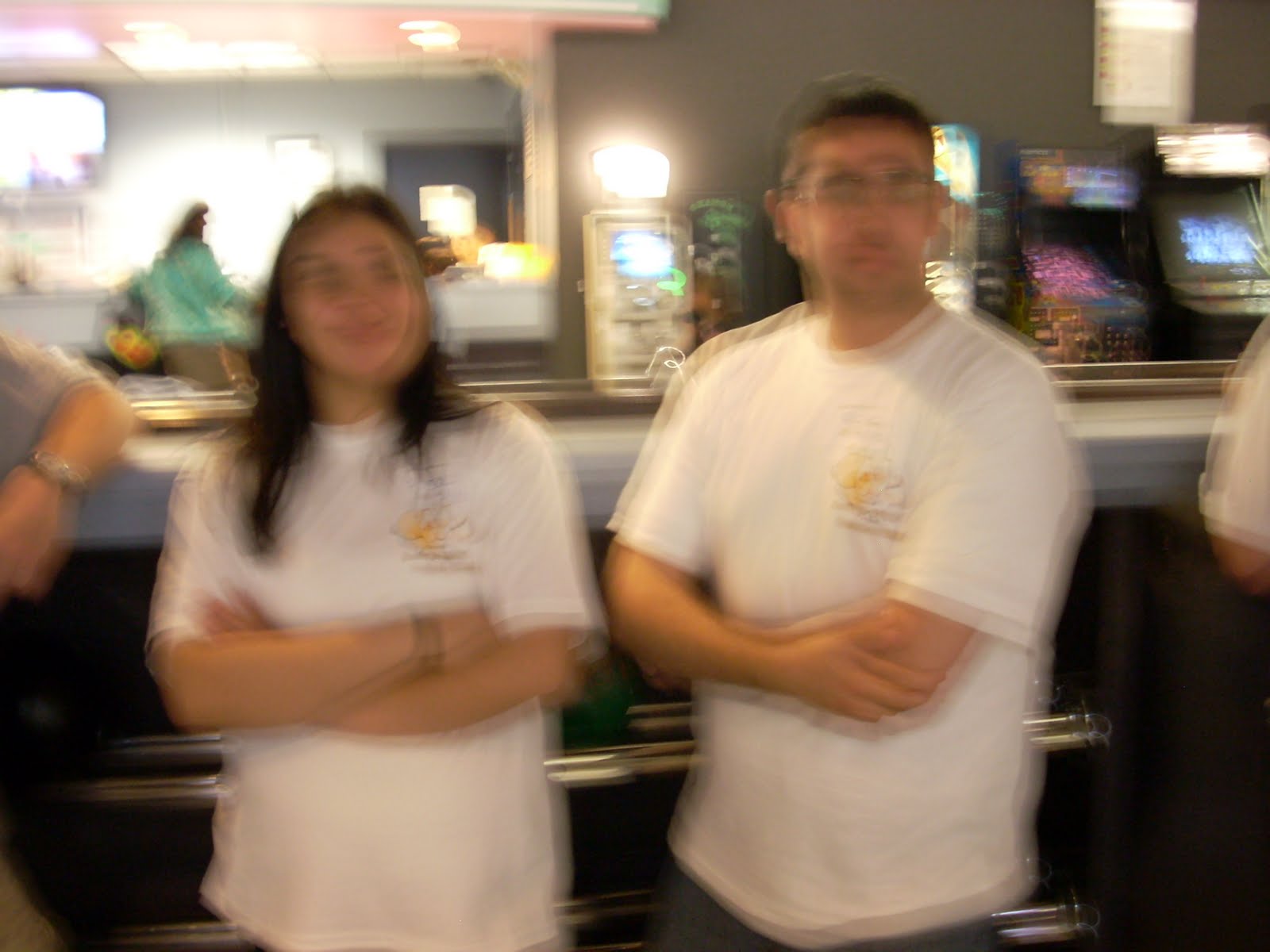In this blurry photograph, a woman and a man stand inside what appears to be an arcade, surrounded by classic video game machines. Both are dressed in white t-shirts featuring a black and yellow design on the top left. The man, who is taller by about a foot, sports short, cropped brown hair and glasses, while the woman has long brown hair. They both have their arms crossed; the woman is smiling slightly, and the man has a neutral expression. Behind them, a woman in a green sweatshirt is visible, along with other people whose arms extend into the frame. The walls in the space are gray, contributing to the overall muted backdrop. Additionally, there is a man with a wristwatch whose arm appears next to the woman on the left.